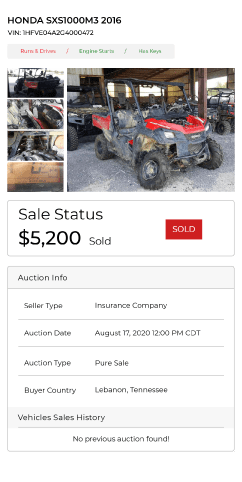The image displays a webpage detailing a 2016 Honda SXS1000M3. At the top, the text "Honda SXS1000M3 2016" is prominently displayed in black print, followed by the Vehicle Identification Number (VIN). Below this, a gray banner features slightly blurred red text that appears to read "RURN Drivers." In green print, the banner also states "Engine Starts, Ends, Has Keys."

The main content area is set against a white background and includes several images. On the right side, a larger image showcases a red side-by-side vehicle with a black frame and wheels, where the front right wheel noticeably bends inward. Adjacent to this, smaller images in panels show various angles of the vehicle. One of these images depicts another side-by-side vehicle in a camouflage pattern, highlighting just the front part. The cement ground beneath these vehicles is visible, and another similar outdoor recreational vehicle is shown in a separate panel.

Towards the bottom of the webpage, the sales status is indicated, showing a price of $5,200. A red square with white text inside prominently displays the word "SOLD."